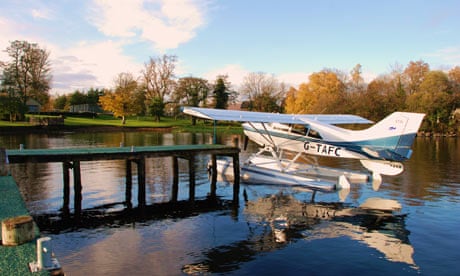In this blurry, portrait-mode photograph, a seaplane is captured as it prepares to land on a small, still lake. The top third of the image features a light blue sky adorned with white clouds on the left. This is followed by a strip of autumnal trees displaying greens, oranges, and yellows. The lake's water starts out dark, offering a mirror image of the scene above, then transitions to a lighter blue towards the bottom right corner. The seaplane, marked with the call letters G-TAFC, is primarily white with a large aqua stripe running along its body and tail. Its reflection is clearly visible in the tranquil water. On the bottom left-hand side of the photograph, a portion of a green docking area can be seen, complete with a docking structure. The overall scene captures a peaceful moment in nature with the serene ambiance of a beautiful day.